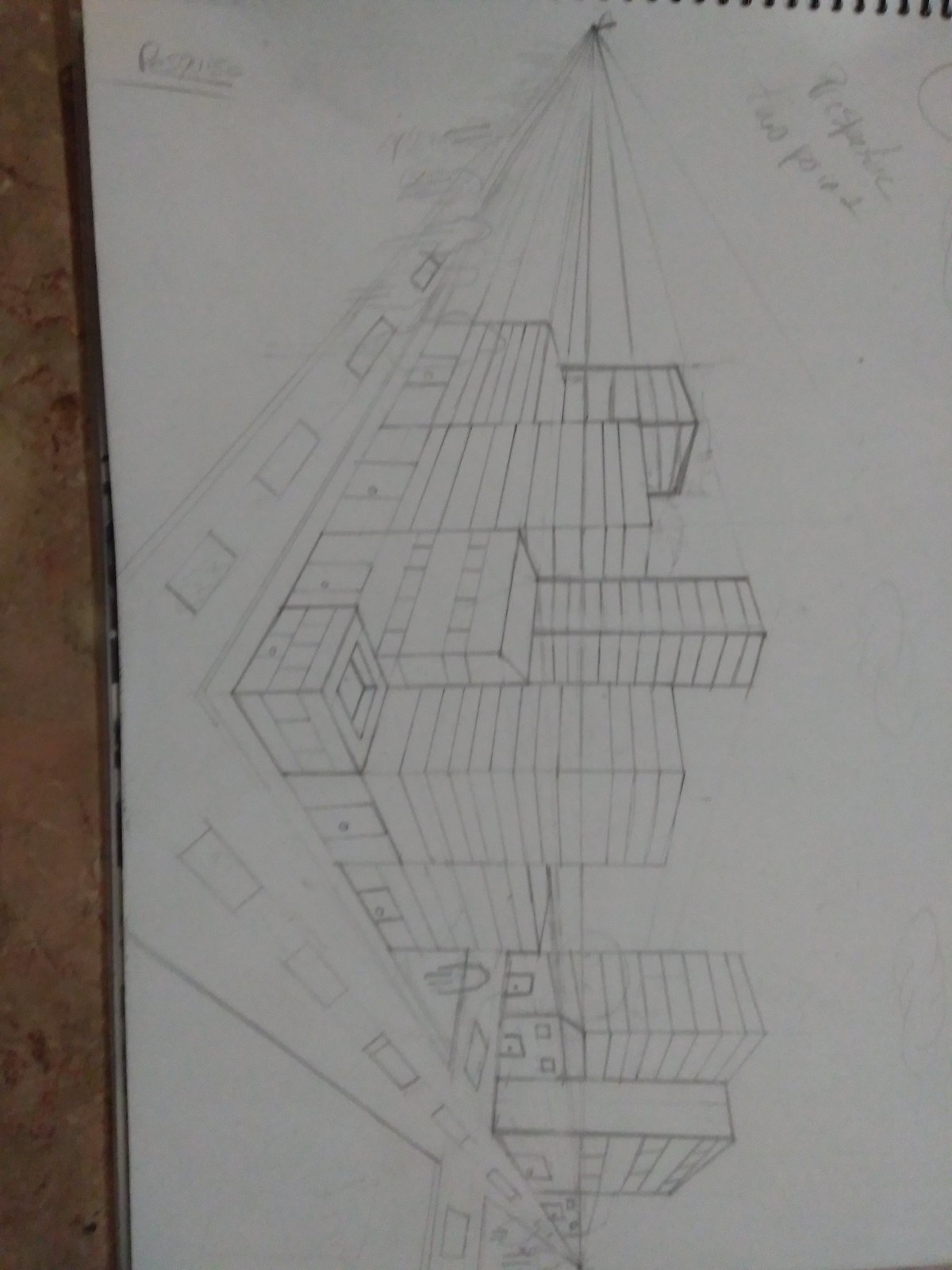A meticulously detailed pencil drawing on white paper, positioned sideways, portraying an urban landscape reminiscent of a metro park. Dominating the scene are numerous towering skyscrapers interspersed with shorter buildings, illustrating how a cluster of structures can create a village-like atmosphere within a city. Nestled inconspicuously between two high-rises is a solitary house, adding a quaint contrast to the modern surroundings. The streets are dotted with what appear to be cars, though their indistinct form leaves some ambiguity. One of the skyscrapers stands out with its darker pencil shading, adding depth and perspective to the drawing. The viewpoint suggests an observer's perspective from within a car, evident by a rust-colored hue at the bottom of the image. Despite the bustling environment, the streets are peculiarly devoid of people, evoking a sense of stillness and solitude in an otherwise lively setting.